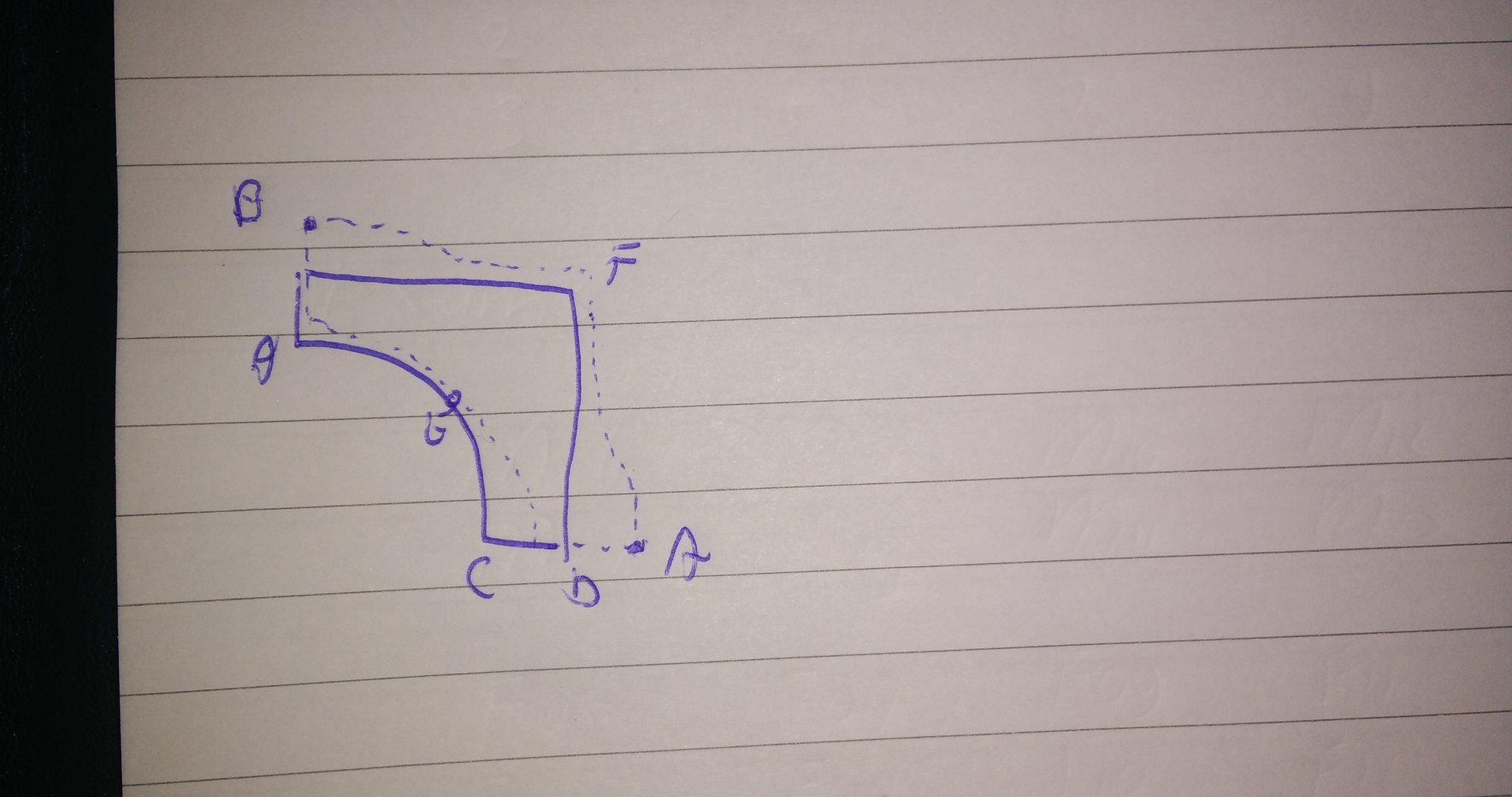The image displays a geometric figure illustrated with blue ink. The primary figure is a solid path that starts as a vertical line extending upwards. At the top, the line takes a sharp 90-degree angle turn to the left. It continues horizontally before taking another 90-degree turn and descends slightly. Following this, the line makes a right turn at another 90 degrees, moving back to the right. It then curves downwards, forming a semi-circular arc until it is vertically aligned in a downward direction. Subsequently, it takes a final 90-degree turn to the right and meets the initial vertical line. The corners of this shape are annotated with letters.

Adjacent to this solid figure, and slightly shifted upward and to the right, there is a similar shape depicted with dotted lines. This dotted shape closely mirrors the original solid shape but is offset just enough to create a clearer distinction between the two forms.